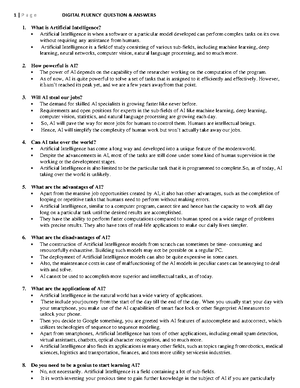This image showcases a blurry, black and white document titled "Digital Fluency Questions and Answers." The content is arranged in an outline format featuring eight questions, each presented in bold black text. Below each question, there are bullet points listing the answers—ranging from two to four per question. Despite the proximity or distance from the viewer, the text remains illegible.